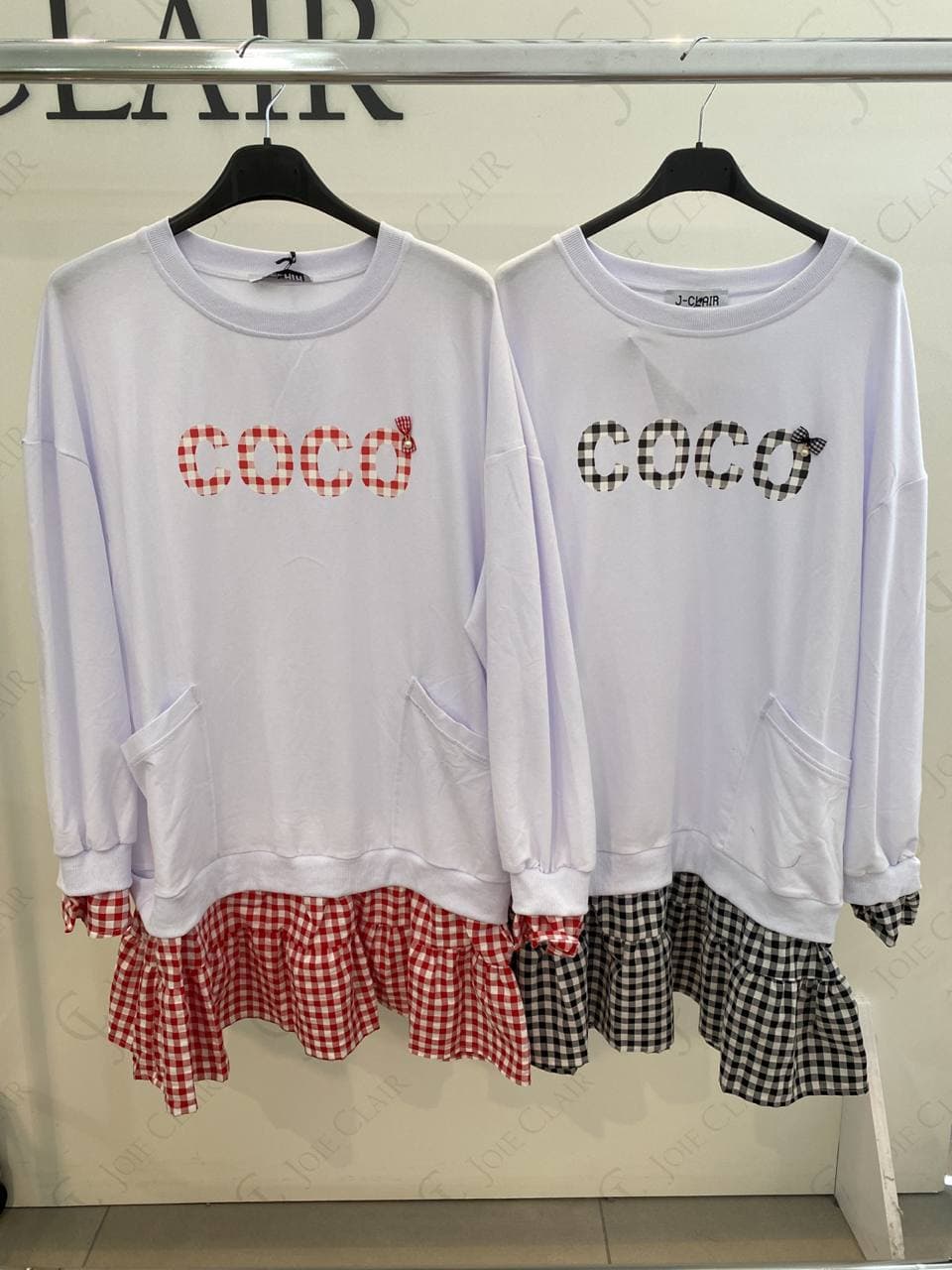The image depicts two intricately designed garments hanging side-by-side on a bar rack, each on its own black hanger. These handmade, sweatshirt-like tops have been creatively transformed into mini dresses, complete with matching ruffled bottoms. One set features a white sweatshirt with added red and white gingham ruffle at the hem and cuffs, while the other mirrors the design in black and white gingham. Both sweatshirts have "COCO" embrodiered across the front in coordinating gingham fabric, with a charming little bow finishing off the "O". The black and white version is on the left, and the red and white version is on the right. The garments, with their pockets and chic gingham details, are displayed in a minimalist white-walled space, giving off an inviting boutique vibe. The partial word "CLAIR" is visible behind them, suggesting the name of a store or brand. These matching sets exude a cute, cohesive style, making them appear perfect for sibling outfits or a charming marketplace listing.